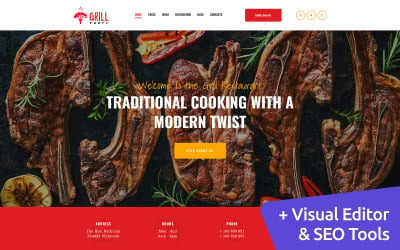Welcome to the Grill Restaurant: Traditional Cooking with a Modern Twist. The center of our homepage showcases a vibrant, high-quality image featuring five chunky pieces of perfectly grilled meat, surrounded by a colorful array of vegetables. The meats are cooked to perfection, with a tantalizing char on the outside, promising a burst of flavors. The background sets a rustic yet contemporary ambiance, enhancing the visual appeal with hues of red, brown, green, blue, white, and yellow from the fresh vegetables. At the bottom right, you'll find handy tools such as a visual editor and SEO options, ensuring an optimal browsing experience.